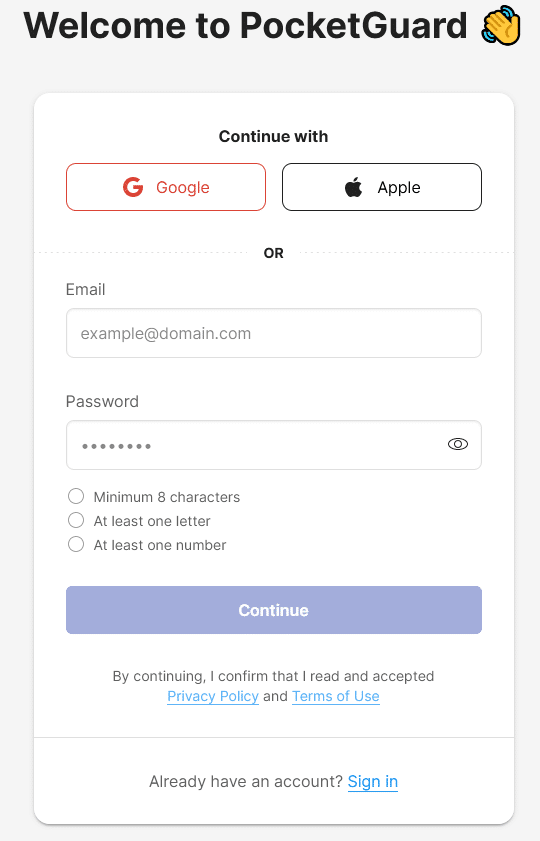The screenshot depicts the welcome screen for the PocketGuard app. At the top, the text "Welcome to PocketGuard" is prominently displayed alongside a waving hand emoji. Below this, users are given options to continue with Google, Apple, or email. The email input field shows "example@domain.com," followed by a password input field represented with several dots, symbolizing hidden characters. An eye icon is present to the right of this password bar, presumably to reveal the entered characters. The password criteria listed include a minimum of eight characters with at least one letter and one number. The screen also features continued action buttons and a statement confirming that by continuing, the user agrees to the privacy policy and terms of use. There is also a prompt for existing users to sign in. The image is portrait-oriented and solely consists of UI elements without any people, animals, plants, buildings, vehicles, or landscapes.